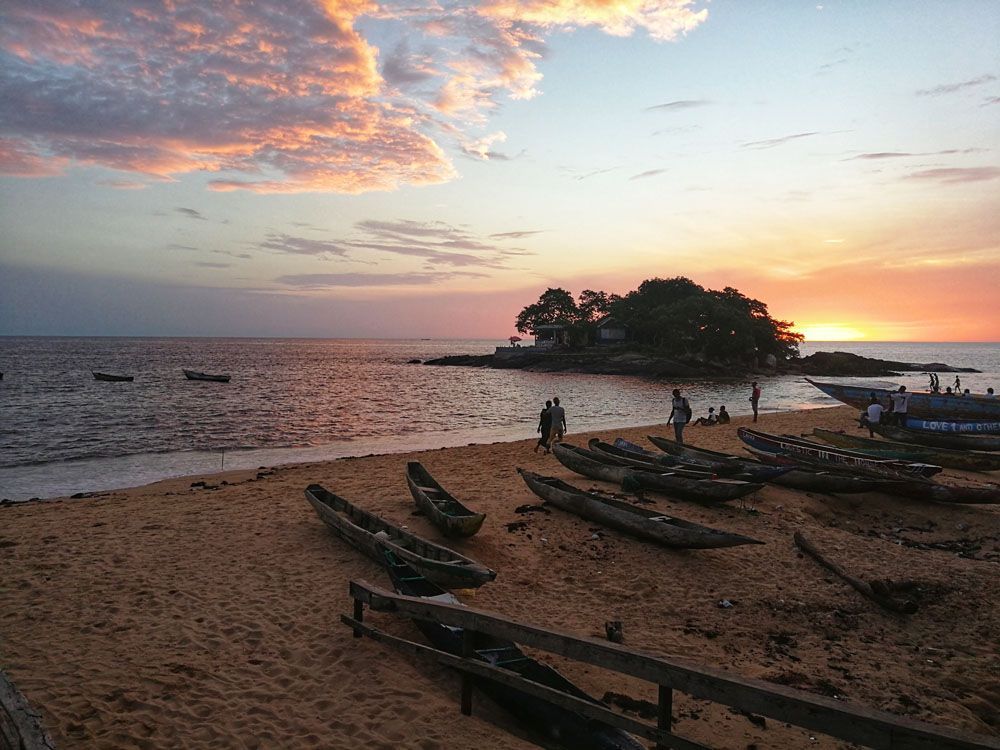As the sun sets over the tranquil sea, the sky is a masterpiece of light blue transitioning to soft peaches, light yellows, and hints of purple, with pink and purple clouds high on the left. Along the orangey-colored sandy beach, approximately twelve people meander and relax, with a noticeable scattering of trash and a railing extending from the bottom right towards the water. About ten beached kayaks, with two more floating near the shore, suggest a day of fishing. To the right, an almost silhouetted small island stands, marked only by the dark shapes of trees and possible homes. The water itself, gently undulating, completes the serene and picturesque scene.